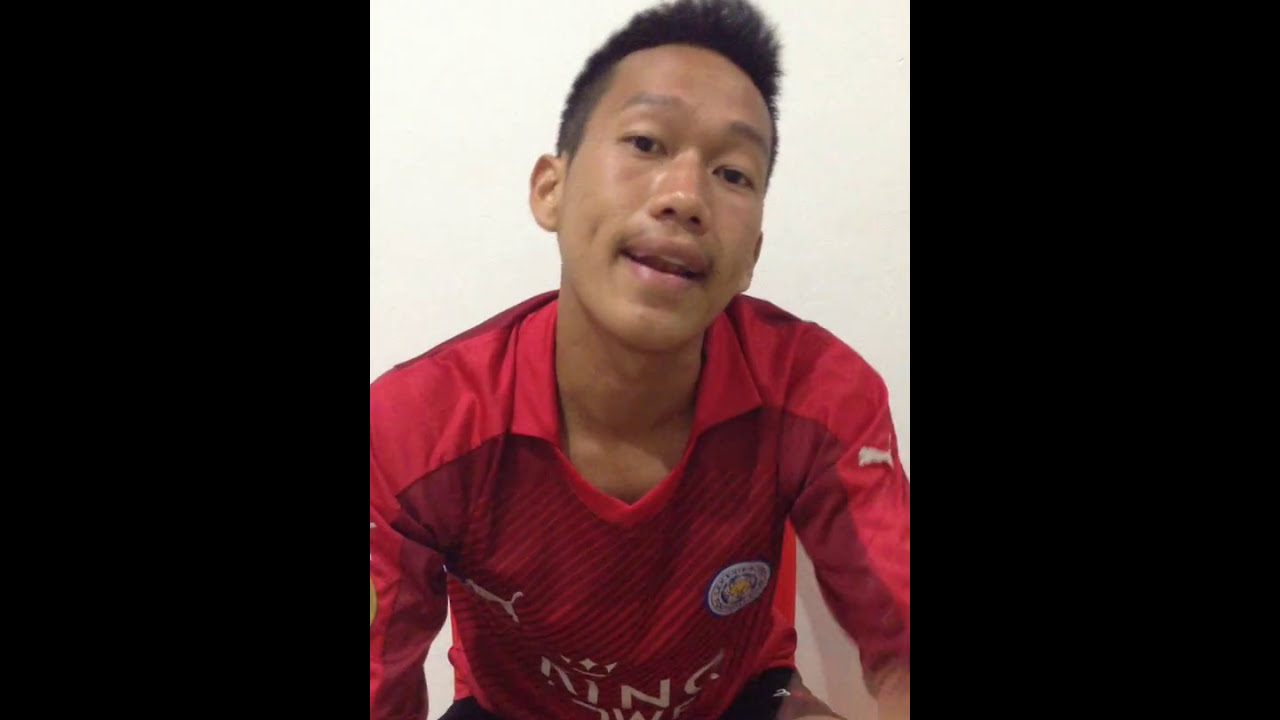This is a detailed photograph of a confident young Asian man, potentially in his early 20s, exhibiting a cocky demeanor. He is wearing a distinctive red Puma jersey adorned with a white Puma logo on the left side of his chest and on his sleeve. The jersey has a collar, and written across it in white text is the word "King," with a crown over the 'i'. The man has short black hair on the sides and spiky hair at the front, coupled with dimples on his cheeks that suggest a slight smile or mid-sentence expression. 

He appears to be leaning slightly forward, looking directly into the camera with his face tilted slightly to the right, giving off an air of assuredness. The background features a light beige wall, flanked by black bars on both sides of the image. The setting is a well-lit indoor space. The man's engaging expression and pronounced facial features, along with the sporty attire, point towards him possibly playing a professional sport, likely soccer, given the branding on his shirt.